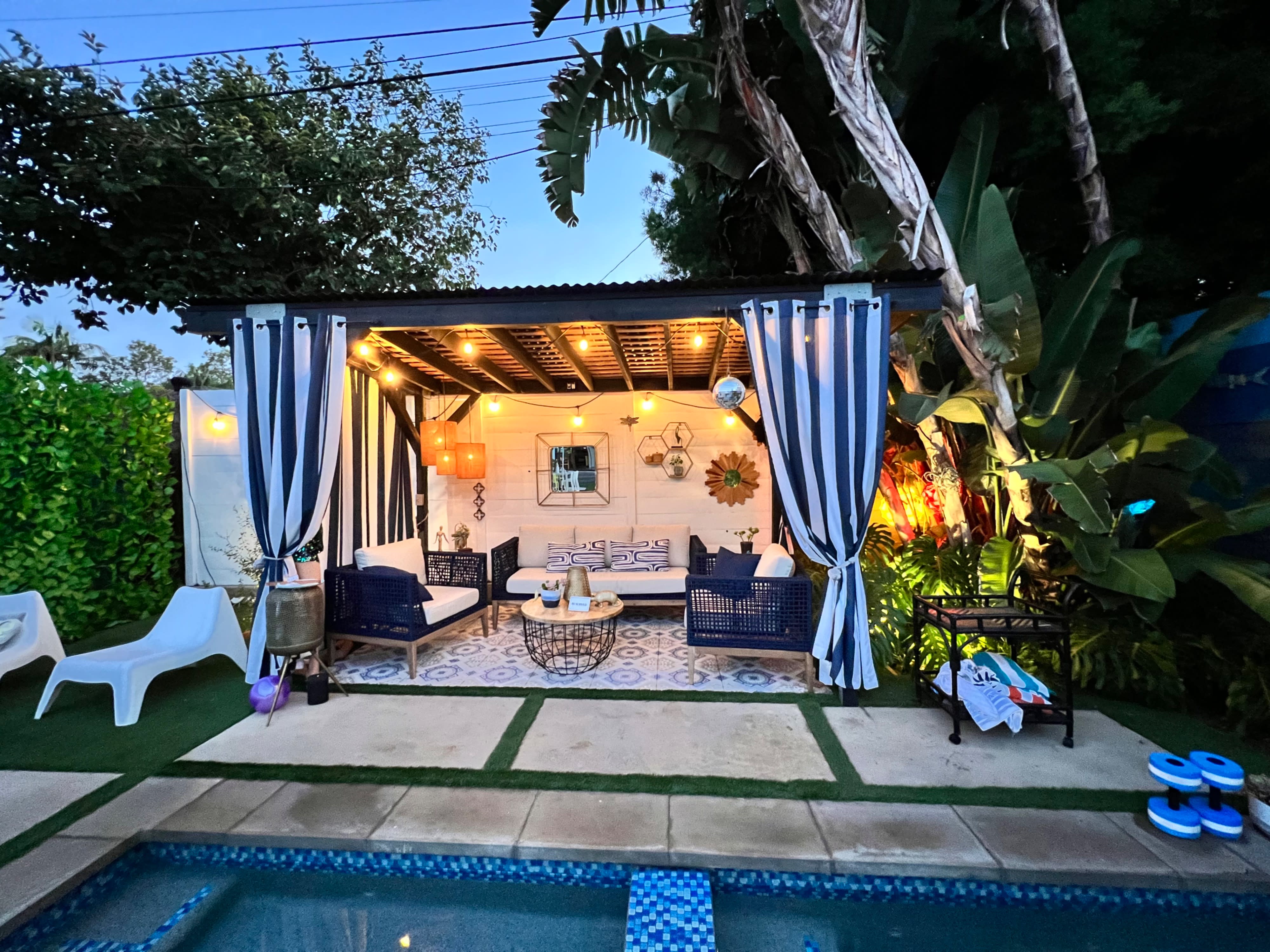The image captures a cozy and inviting outdoor poolside patio that exudes warmth and relaxation. This small backyard setup features a cabana next to a shimmering swimming pool adorned with blue, light blue, and white mosaic tiles, giving the water a beautiful, intricate pattern. Surrounding the pool, there are rectangular cement squares interspersed with patches of grass, adding a touch of green to the overall decor.

The cabana itself is thoughtfully decorated with navy blue and white drapes that match nicely with the patio's furnishing and the white walls. Inside the cabana, there's a collection of comfortable seating, including several navy blue and white couches, as well as a plush white sofa adorned with uniquely patterned black and white pillows. A table is centrally placed among the seating, creating a perfect spot for relaxation or social gatherings.

The ambiance is further enhanced by the warm shades of yellow and orange emanating from numerous large fairy lights, casting a gentle glow over the entire area. On the ground, you can see white and blue patterned tiles adding to the aesthetic harmony of the place. The patio also features white lounge chairs to the side, perfect for basking in the sun. Near the bottom right corner of the image, two water weights rest, possibly for pool exercises.

This outdoor room is completed with honeycomb-style wall décor and a backdrop of lush trees under a clear sky, making it an ideal retreat for reading, resting, or enjoying a cheerful gathering. The overall vibe is inviting and fanciful, evoking a sense of comfort and refined aesthetic.